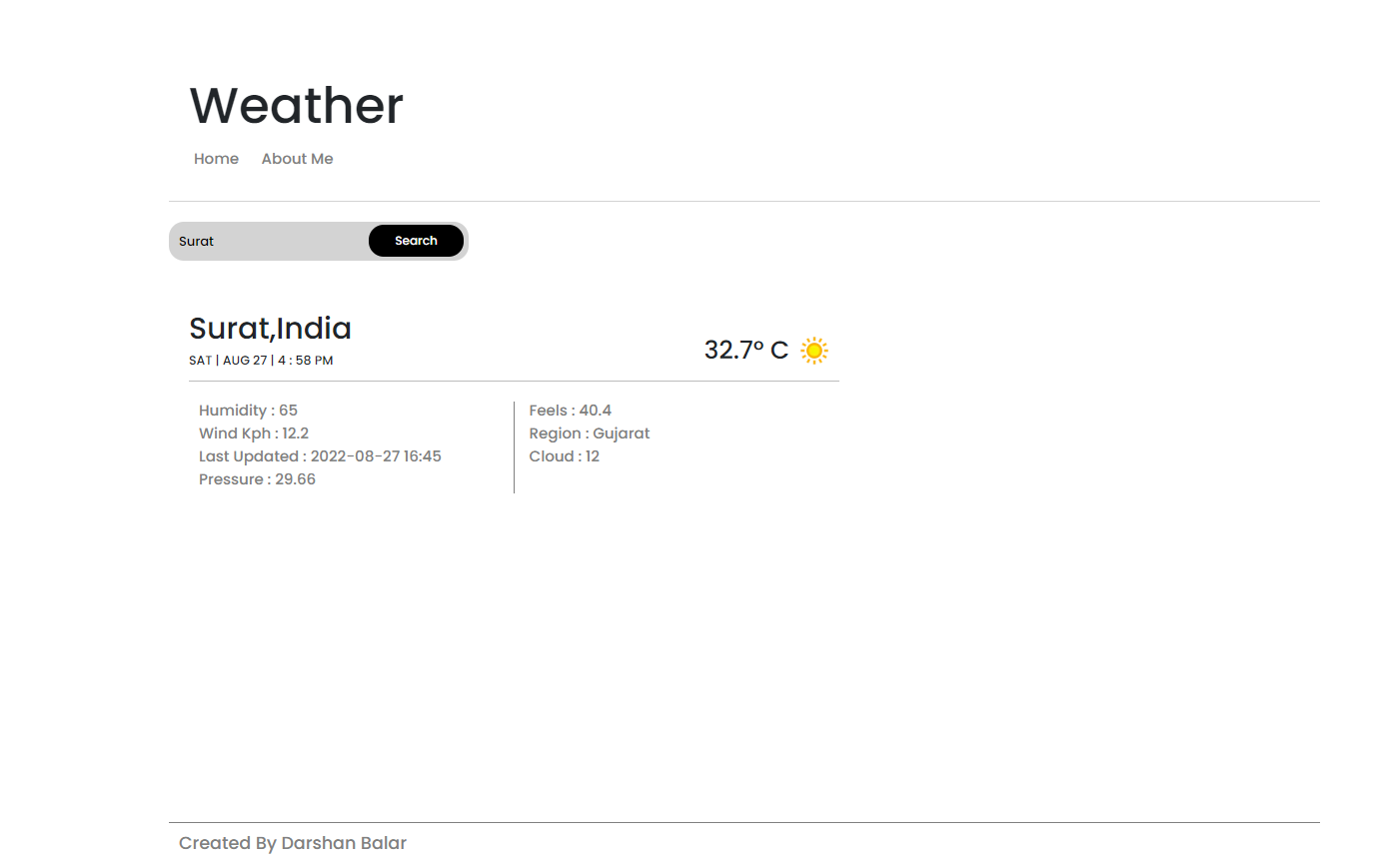The image features a predominantly white background. In the upper left corner, the word "Weather" is prominently displayed in black, serving as the main header. Directly beneath this header are navigation links labeled "Home" and "About Me," separated by a gray horizontal line.

Below the navigation bar, the name "Surat" is prominently featured in a large font, with a gray search data field immediately next to it. To the right of this field is a black search button with the word "Search" displayed in white font.

Further down on the page, the text reads: "Surat, India, Saturday, August 27th, 4:58 p.m." To the right of this text, the temperature is displayed as "32.7 degrees Celsius" accompanied by a yellow sun icon. Below this information is another horizontal line.

Underneath the line, a detailed weather report is provided: 
- Humidity: 65%
- Wind: 12.2 kph
- Last Update: 2022-08-27 16:45
- Pressure: 29.66

A vertical line separates the next section. On the far right, additional details are listed:
- Feels like: 48.4 degrees
- Region: Gujarat
- Cloud coverage: 12%

There is considerable white space throughout the image, providing a clean and uncluttered appearance. Another gray horizontal line separates the main content from the footer, which credits the creator: "Created by Darshan Balar."

The color scheme of the image is primarily white, with accents of black, gray, and yellow.